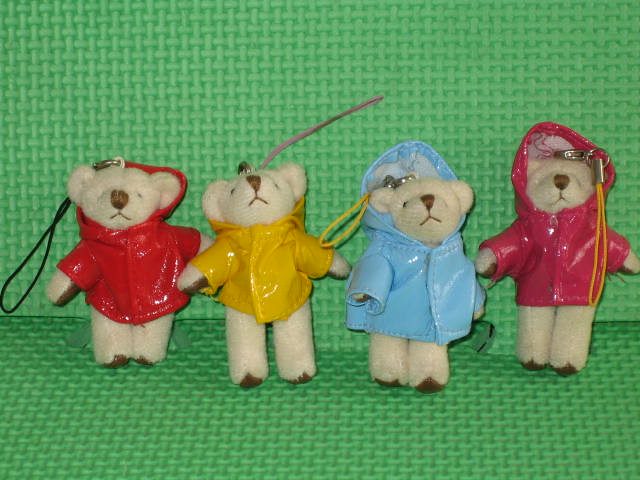The photograph features four small, beige-colored toy bears that appear to function as keychains. Each bear is crafted from cloth fabric and has brown thread detailing for the eyes, nose, and mouth. They are lined up side-by-side, neatly leaning against a green puzzle mat that serves as both the floor and the backdrop of the image. Each bear is adorned in a different colored raincoat; starting from the left, they wear red, yellow, light blue, and pinkish-red garments. From the top of their heads, loops attached to clasps can be seen, from which colored strings dangle: black on the first bear, pink on the second, and yellow on both the third and fourth bears. This detailed setup suggests a display-like arrangement, emphasizing the multicolored theme and the playful setting with the puzzle mat background.